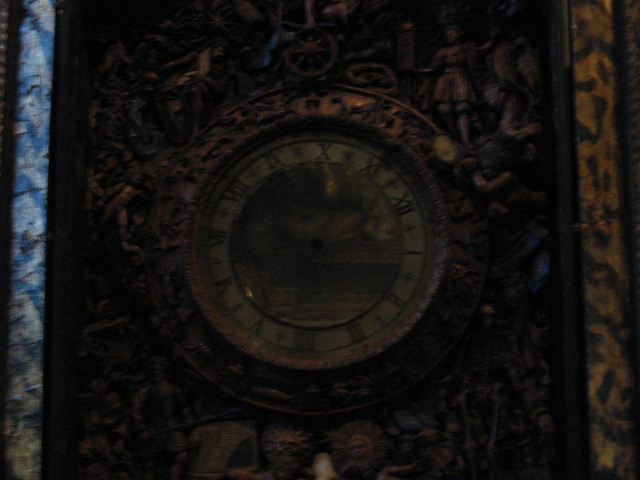The image showcases an old, grainy, and ornate circular wall clock with a heavily carved wooden frame. The outer frame, rich brown in color, is intricately adorned with various figures, including numerous people, a skeleton, a cartwheel, and multiple sun faces. The frame forms a rectangular shape around the circular clock. The clock itself has a dark, central hole where the hands are missing, and its inset is a greenish-grey shade. The face of the clock is white, set beneath glass and features Roman numerals, with XII at the top, VI at the bottom, and IV on the bottom right, creating the structured timepiece. To the left side of the clock, there is a blue and white ceramic tiled area, and to the right, there is a dark brown and black tiled area. The image is characterized by a lack of light, contributing to its overall dark and antique appearance.